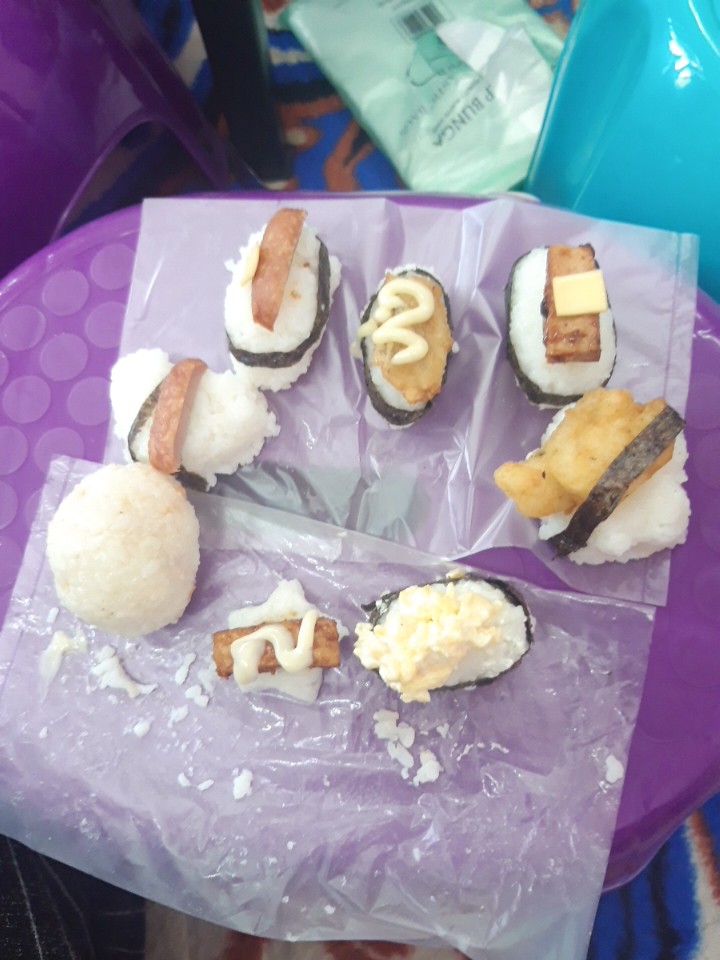The photograph features an assortment of homemade sushi artfully displayed on two pieces of parchment paper, which are laid atop a vibrant purple stool, subtly adorned with polka dots, serving as a makeshift table. The sushi pieces are an eclectic mix characterized by unconventional toppings. Starting from the bottom left and moving clockwise, the first piece is a simple ball of rice. Next is a ball of rice wrapped in black seaweed. Following this is a star-shaped rice piece with a brown topping, drizzled with white mayo-like sauce. There are several sushi configurations containing rice topped with elements such as canned meat (likely Spam), fish sticks, and chicken nuggets, some of which are secured with seaweed bands. Overall, there are around seven to eight pieces in total, presenting a spectrum of colors and textures, from beige and brown to red and yellow. The background reveals additional objects adding context, including glimpses of a chair leg in black, another possibly blue chair, and a package with blue writing and a barcode.